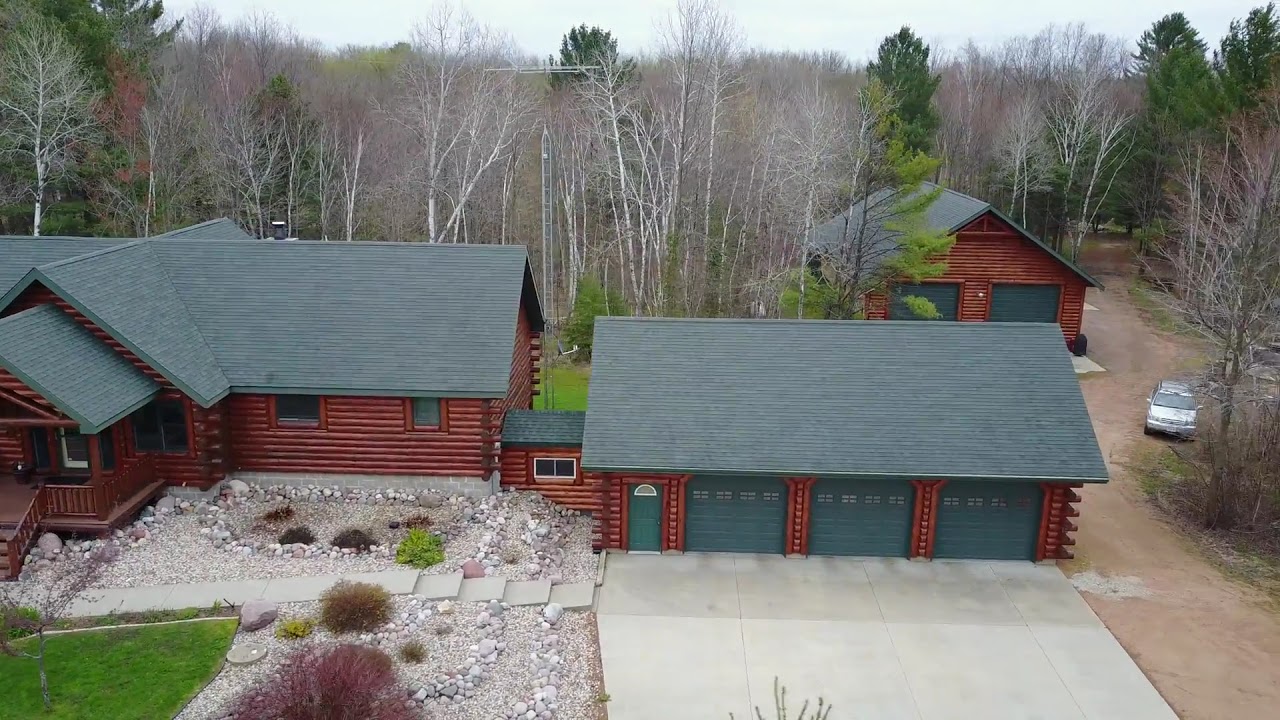The aerial view highlights a picturesque outdoor setting under a light, grey sky. Dominating the scene are tall trees, some stark white and leafless, juxtaposed with a few fully green-leaved counterparts. Central to the image is a sprawling log cabin with rich maroon-red logs, whose left side, featuring a wide porch with green triangular roofs, is cut off at the entryway. To the right of the cabin sits a three-stall garage, also constructed from logs and adorned with teal doors and a green tiled roof. Adjacent to this garage stands another log building, smaller with two large green doors. Behind these structures lies a pole barn with matching green roofs and two large garage doors. The foreground reveals a mix of rocky terrain and a small patch of green lawn towards the bottom left, enhancing the rustic charm of this serene woodland retreat. A silver car is parked on the concrete driveway area to the right, which extends towards the pole barn.